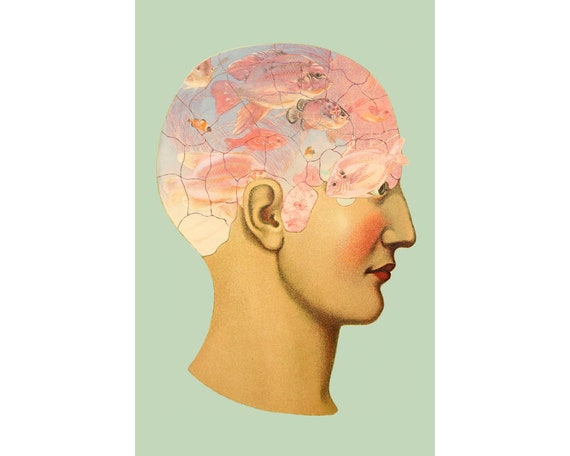This digital illustration features a side profile of a bald human head, turned with the nose facing the right side of the image. The person has olive-colored skin with pearly peach blush and red lipstick, suggesting a feminine appearance. The background is a light olive green hue. The top half of the head is depicted as if it were a jigsaw puzzle, with sections resembling the compartments of a brain or skull. Instead of brain matter, the segmented area contains pink fish swimming in blue-gray water, evoking the image of a fish tank. The entire scene conveys a surreal and artistic style reminiscent of classic 17th or 18th-century portraiture.